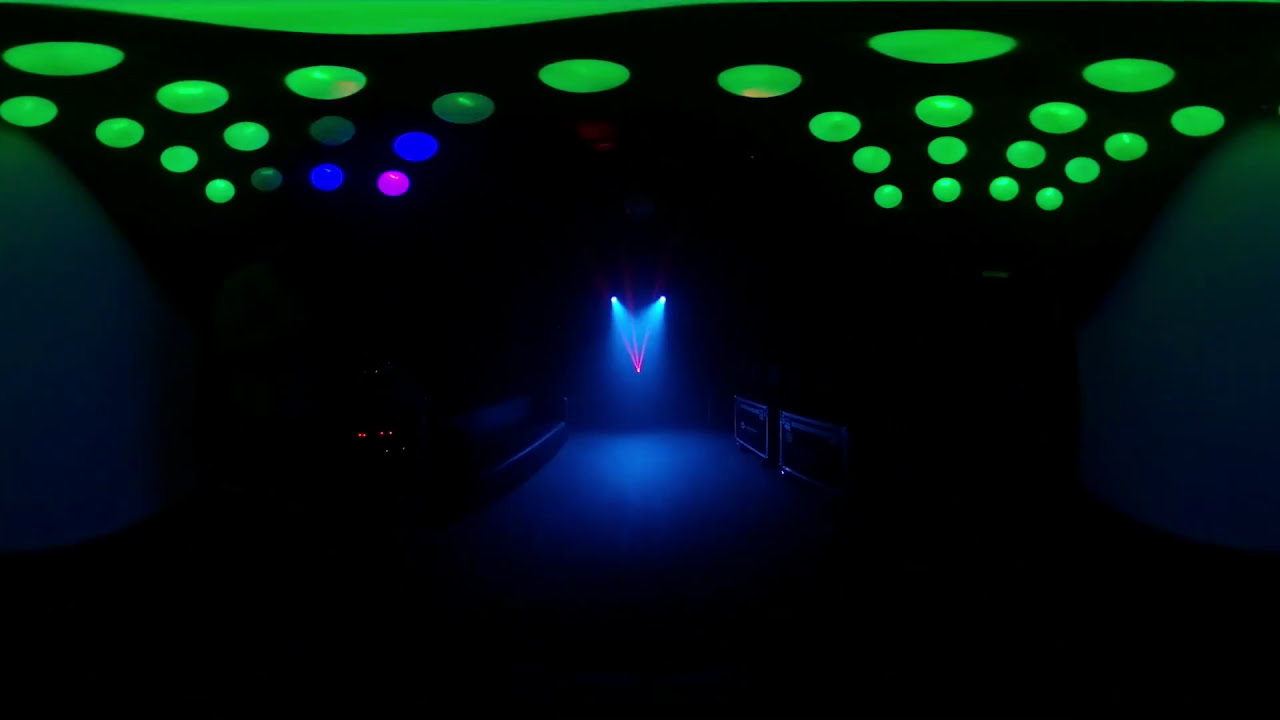The image depicts a computer-generated environment, likely a virtual reality space, characterized by its distinctly dark and vibrant atmosphere. The room is dimly lit, with a noticeable distortion at the top hinting at a 360-degree view. The ceiling features numerous small spherical green lights that add a surreal touch to the scene. Alongside these green lights, there's a scattering of blue, purple, and darker green globes. Dim blue lights faintly illuminate the room, casting a muted blue hue across the space.

On the left side of the image, a leather couch is visible, while on the right, there are black and silver crates with a blue tint from the lighting—these crates resemble those used for transporting music equipment, suggesting the space might be a concert green room or staging area. Central to the scene is a set of three red, laser-like lights arranged in an upward-branching formation. Below them, blue spotlights create a faint pathway, punctuated by intermittent red lights. The overall environment is highly colorful and artificial, contributing to an unusual and vividly detailed visual experience.